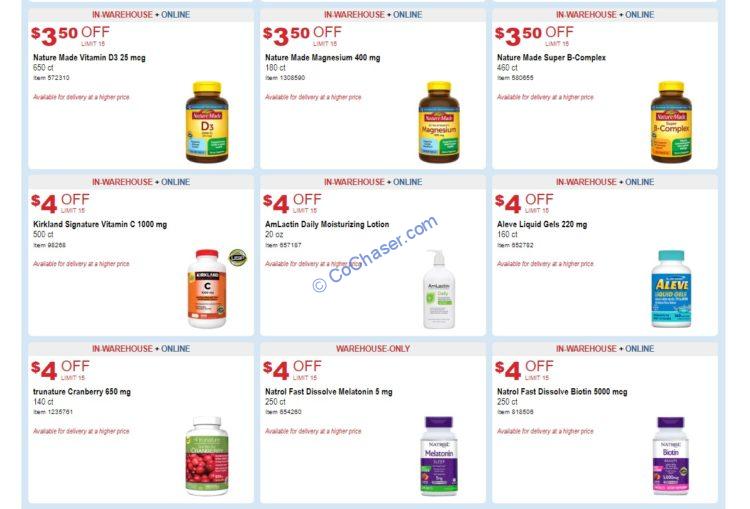This image, sourced from cogchaser.com, showcases the weekly sales flyer for CVS Pharmacy. It prominently features nine over-the-counter vitamin products arranged in a grid format, with three products per row and column. Each product is displayed against a clean white background, making the item details easily distinguishable. The discounts, highlighted in red font, range from $3 to $4 off per item, with the cheapest discount being $3.50 off and the highest at $4 off. The product names, quantities, and sizes are clearly listed in black font. In the lower corner of each product depiction, subtle red print indicates the expiration date of the sale. The meticulous layout focuses solely on the sale items, ensuring all pertinent details such as pricing and specifications are front and center for the viewer.